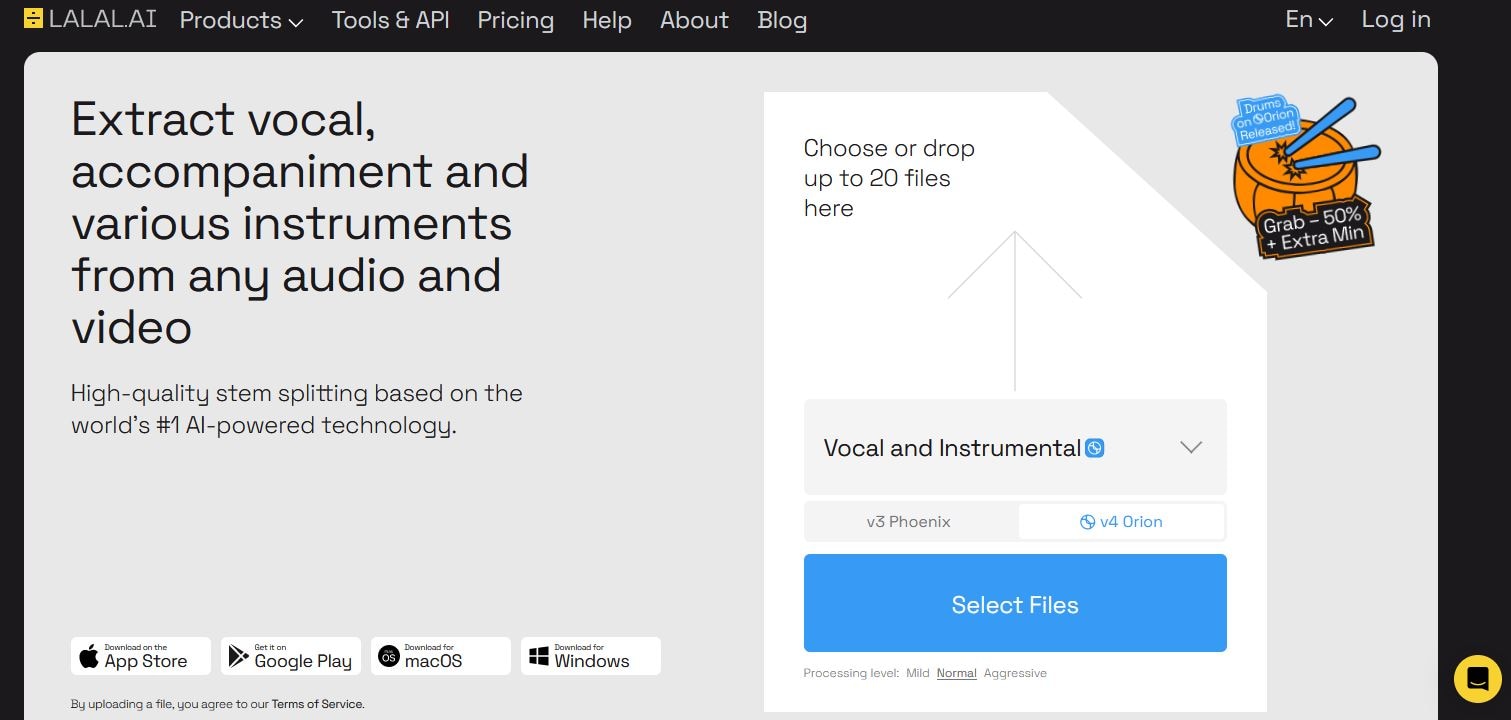Here's a clean and detailed caption for the image described:

---

**Screenshot Description:**

The screenshot captures the homepage of a website, identifiable by the header which reads "LALAL.AI". The navigation bar at the top includes links labeled "Products" (with a dropdown menu), "Tools and API", "Pricing", "Help", "About", and "Blog". On the far right of the header, there's a language selection dropdown labeled "EN" and a "Login" button.

The central area of the page features a service offering that states: "Extract vocal, accompaniment, and various instruments from any audio and video. High-quality stem splitting based on the world's number one AI-powered technology." Below this statement, there is an image of a document with a section that prompts users to "Choose or drop up to 20 files here." Additionally, there are options for stem separation labeled "Vocal and instruments" with a dropdown menu that includes "V3 Phoenix" and "V4 Orion", the latter of which is selected.

A prominent "Select Files" button is located below these options. In the lower right corner of the image, there's a sticker depicting a drum being tapped, with text that reads "Dump on Orion released" and "grab 50% + extra minimum."

Additionally, the bottom right corner features a chat support icon, and a section indicating various platforms where the website's services are available: "Download on the App Store," "Get it on Google Play," "Download for Mac OS," and "Download for Windows."

---